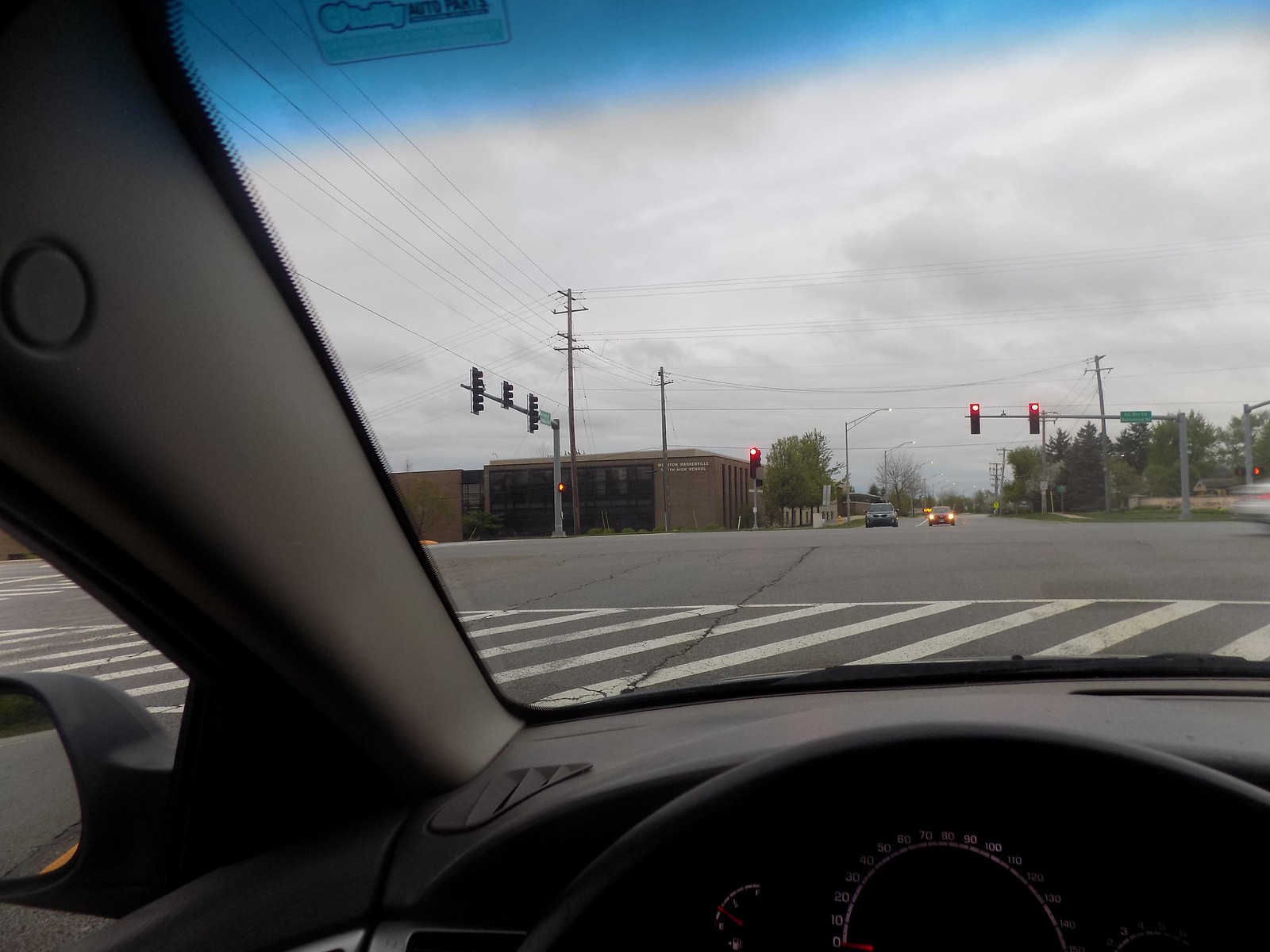The image is a detailed photograph taken from the inside of a car at an intersection in America, as seen from the driver's seat. The dashboard, instrument panel, and part of the steering wheel are visible, with the dashboard being black. The car is stopped at a red light, and outside the windshield, we can see a large open road with a prominent crosswalk painted in diagonal white lines in front of the vehicle. The sky is dark, gray, and heavily overcast, suggesting a gloomy and cloudy day.

On either side of the road, there are telephone poles and wires running across the intersection, and some trees add a touch of nature to the urban setting. The reflection of the street can be seen in the side mirror, and part of the side window and mirror are also visible. Directly across the street, we see a building, mostly brown with large windows, which looks quite old. Two cars are positioned on the opposite side of the intersection; one has its headlights on and appears to be waiting to proceed. Another car is driving away while another approaches, contributing to the sense of a busy, albeit paused, moment at this sizable intersection.